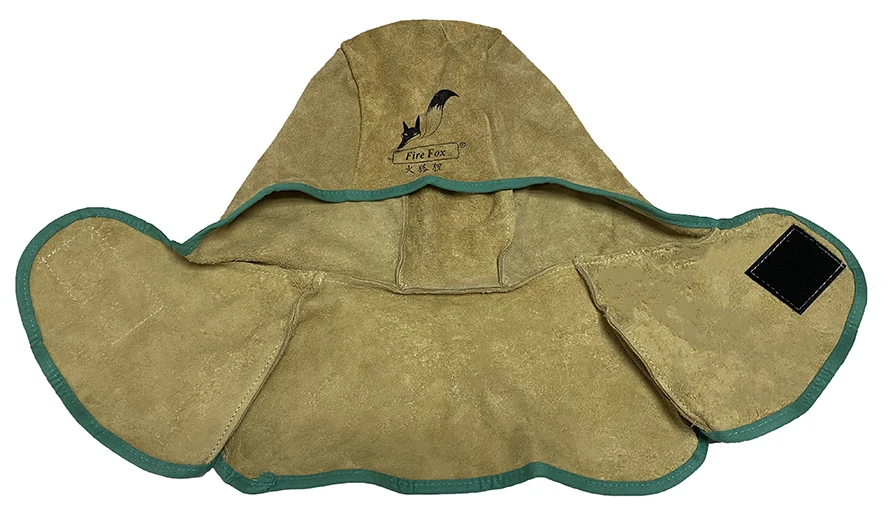The photograph features a brown leather hat with a distinctive green trim around its edges. The hat, designed to strap securely under the chin with Velcro patches on either side, is spread out and flat against a plain white background, showcasing its ear coverings and structure. Prominently displayed on the front of the hat’s hood is a logo featuring a stylized black fox with outlined sections indicating its orange and white fur. Beneath the fox, inside a box, are the words "Fire Fox" in black text, accompanied by Japanese characters. This detailed yet simple image highlights the hat's functional and protective design, suitable for weathering the elements.